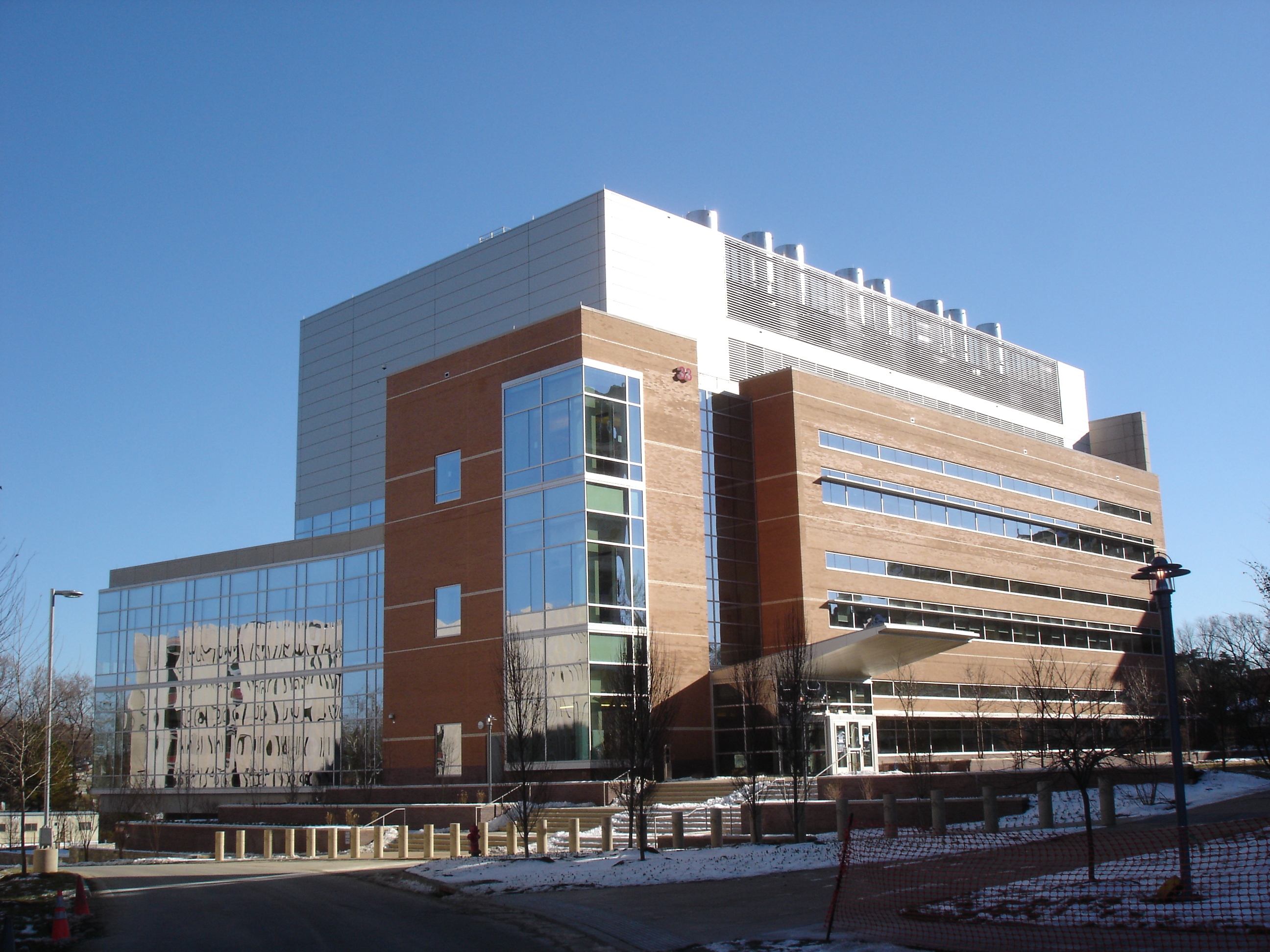This color photograph features a large, multi-story building that resembles a hospital or office complex, centrally positioned against a backdrop of a clear, blue sky. The building stands on a gray asphalt concrete surface, which is partially lined with white snow. The structure itself is characterized by its blockish, square design, with numerous windows adorning its sides. On the left, the windows are a reflective metallic silvery color, mirroring the blue sky behind them, while those on the right have a grayer hue due to the light's angle, also reflecting the sky. 

The building's exterior combines brown and white elements and includes striking reflective mirror windows, contributing to its modern aesthetic. Descending towards the entrance, a number of steps, covered lightly with some snow, lead into the building. In the immediate foreground, away from the building, a single duck can be seen standing on the snow-dusted ground. The scene subtly suggests winter, with barren, leafless trees and visible snow cover. Moreover, there's an area under construction, marked off with orange and vinyl fencing to keep people away. Despite the winter chill, the walkway leading up to the building appears to have been shoveled clean of snow.